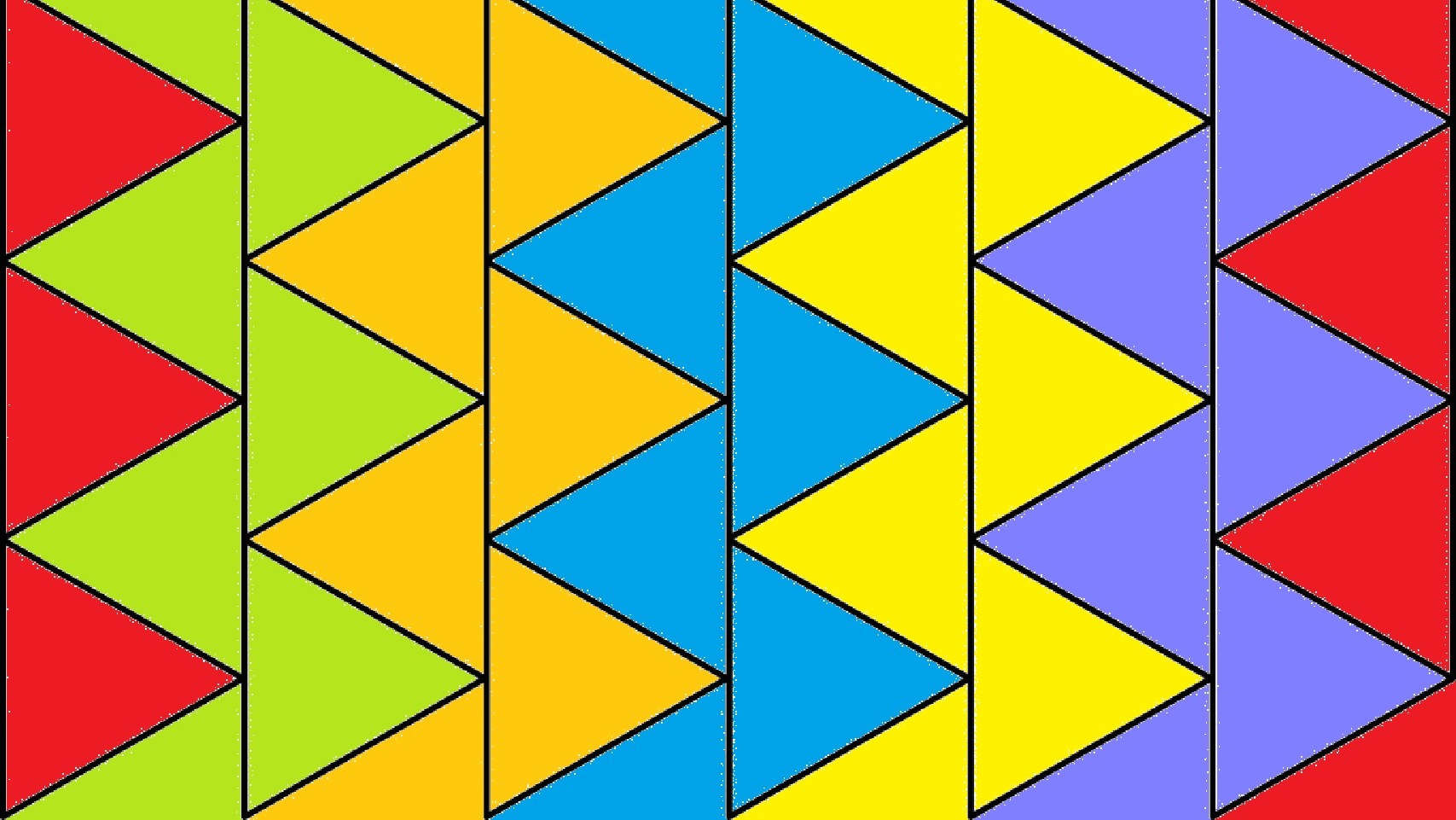The image is a digital artwork featuring a series of geometric-style triangles arranged in a cohesive, interlocking pattern. It consists of six vertical panels, each approximately six to seven inches tall and three to four inches wide, all uniformly sized. The design is characterized by vibrant solid colors and a sequence of zigzag patterns that span across adjoining panels.

Starting from the leftmost panel, it contains red solid triangles that transition into lime green zigzags on the adjacent panel. These lime green zigzags blend into yellow zigzags, which extend halfway into the next panel. The yellow zigzags adjoin with blue triangles, forming blue zigzags that lead into yellow once again. Following this sequence, purple zigzags connect to the yellow, and finally, red triangles reappear, interlocking with the purple ones. Black lines separate each panel, emphasizing the divisions while enhancing the geometric cohesion. All elements are oriented to fit together seamlessly from the sides, creating a fluid, continuous visual flow reminiscent of Art Deco style with the precision and clarity typical of computer-generated imagery.